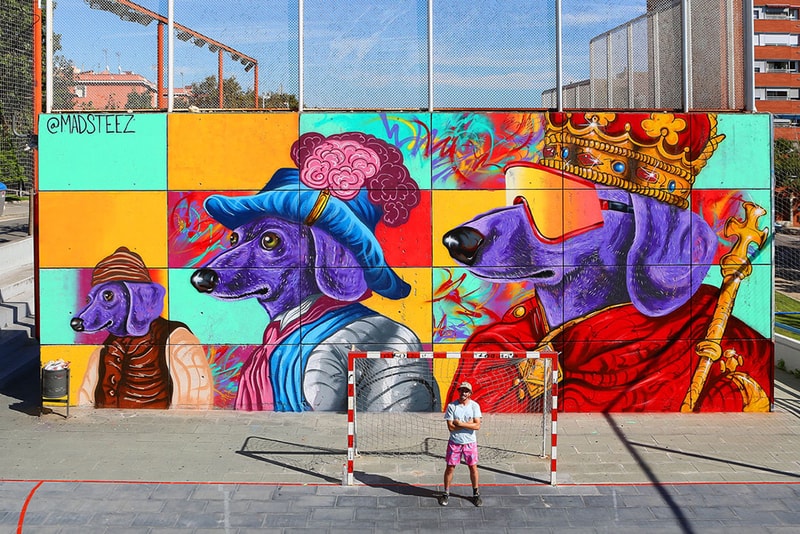The detailed photograph showcases vibrant street art by artist Abmadstiz, or possibly Mad Stills, painted on a large fence within an urban park setting. The mural features an eclectic array of purple and pink dachshunds adorned in various whimsical outfits. At the center, a dachshund sporting a king's crown and sunglasses stands out, exuding a cool, regal vibe. Flanking this "king" are two other playful figures: one dressed in a Three Musketeers-style costume, and another with a more laid-back, stoner aesthetic. In the foreground, a man poses confidently, dressed in pink shorts and a white shirt, accessorized with a hat and sunglasses. He stands before a goal net, likely for soccer or hockey, situated on the stone-paved ground. The scene is lively, colorful, and brimming with creative energy, capturing a moment where street art and urban recreational spaces intersect.